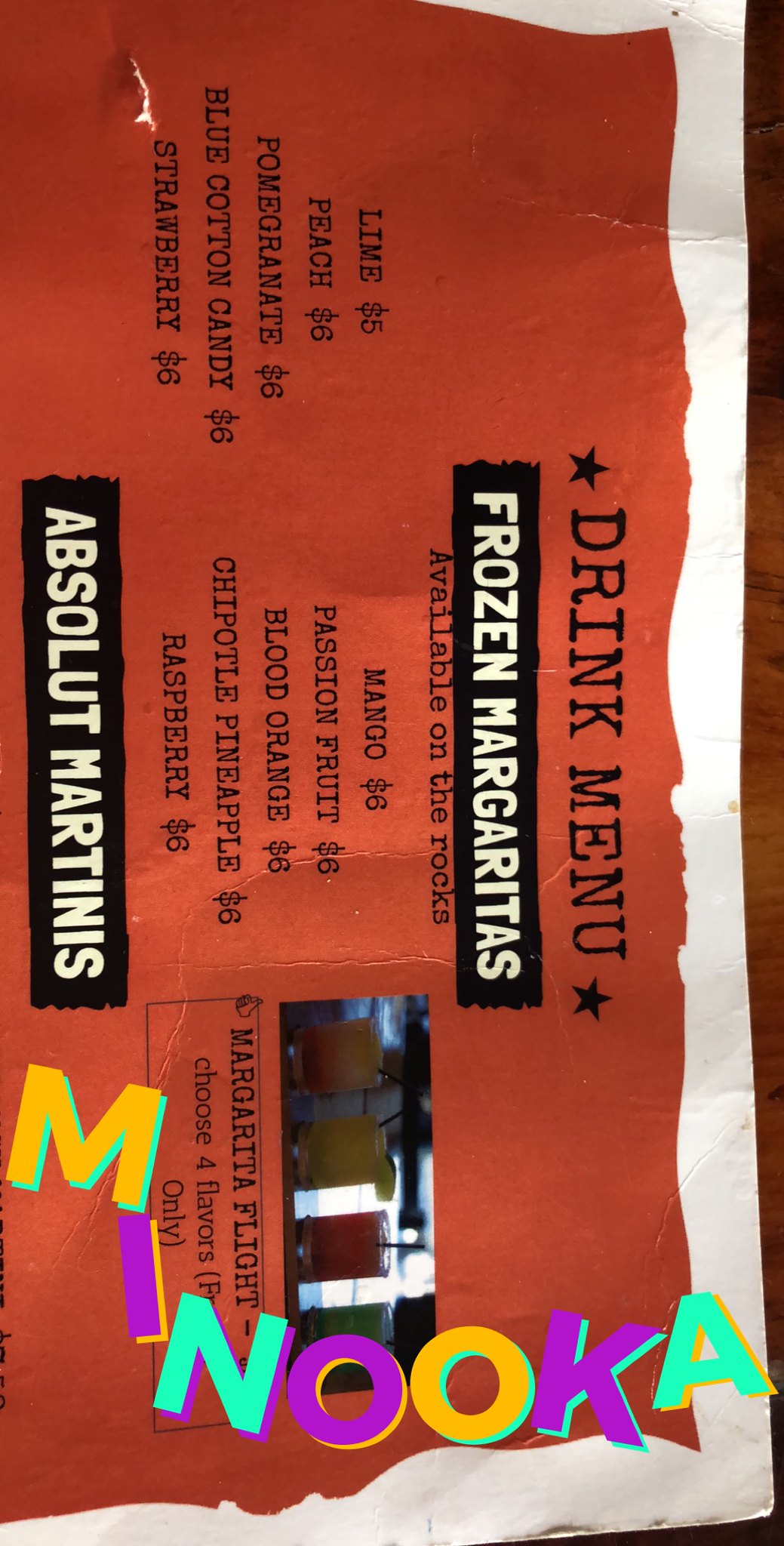This image captures a drink menu displayed vertically, although the photo itself is rotated horizontally, requiring rotation to read properly. The menu, set against a red background with a white border, is titled "Drink Menu" in black font with two black stars flanking the text. Below this, a black rectangle containing the words "Frozen Margaritas" in all capital white font prominently stands out. Directly beneath, in black font, it states "Available on the Rocks". 

The menu is organized into two columns of flavors and prices. The left column lists:
- Lime, $5
- Peach, $6
- Pomegranate, $6
- Blue Cotton Candy, $6
- Strawberry, $6

The right column includes:
- Mango, $6
- Passion Fruit, $6
- Blood Orange, $6
- Chipotle Pineapple, $6
- Raspberry, $6

Additionally, a segment at the bottom in a black rectangle announces "Absolute Martinis". To the right, it offers a "Margarita Flight" option where patrons can choose four flavors, though this text is partially obscured by another item in the photo.

The menu appears somewhat crumpled, suggesting it is a well-used, possibly handheld item, and contains an obscured word starting with "F" followed by "only". The lower part of the image concludes with the text "Minooka."